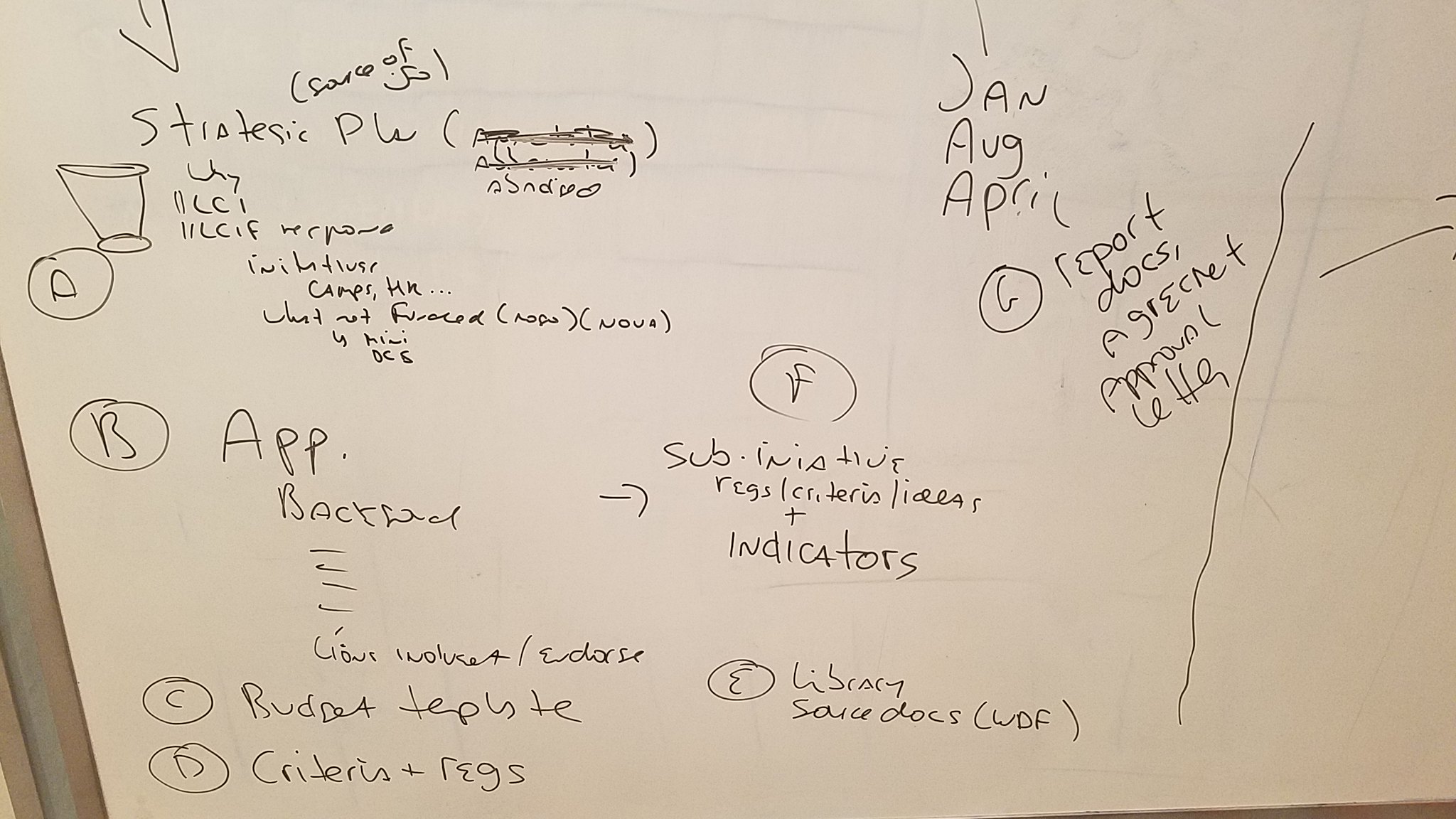The image is a photograph of a whiteboard or poster board densely covered with messy black dry erase marker writing, making it hard to decipher. The board outlines a brainstorming session with various elements categorized and connected by lines, arrows, and zigzag patterns. Prominent features include letters circled from A to G, each followed by respective keywords and phrases:

- (A) App
- (B) Back end
- (C) Budget template
- (D) Criteria + regulations
- (E) Library
- (F) Substantive regulations, criteria, ideas, indicators
- (G) Source docs

Additional notes scattered across the board mention months such as January, August, and April, and terms like "strategize PLS," "statistics," and "report docs, agreement, approval letter." There are also scribbles that are difficult to interpret, further contributing to the chaotic appearance of the board.